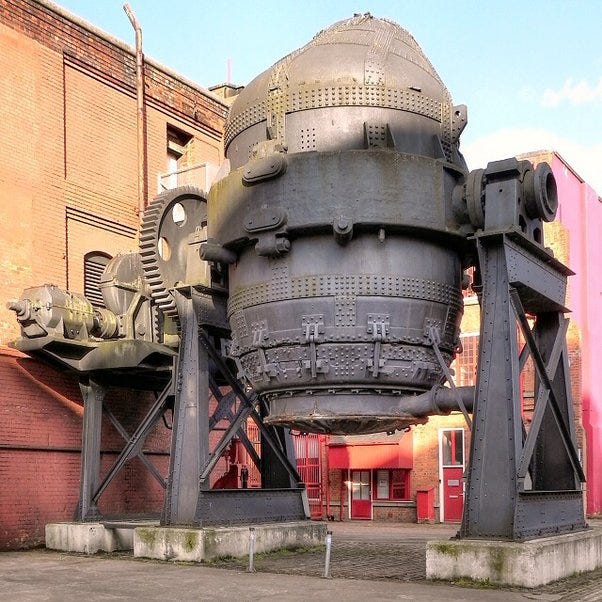The photograph captures a massive, cylindrical steel machine resembling a gigantic metal balloon situated outside a two-story yellow brick factory building. The machine, likely made of iron, is held up by two stone supports connected by metal cross handles. On the left side of the structure, detailed mechanics and a large gear-like apparatus are visible. The machine, dark gray or black in color, rests on a cement sidewalk. The factory building features two red doors on its right side, with a large rectangular glass window above one door and a red trash can placed between them. The building's exterior at the bottom left is painted pink, transitioning to bright pink and yellows as it moves right. The scene is set under a bright daytime sky with white clouds, providing a striking background to the impressive mechanical structure.